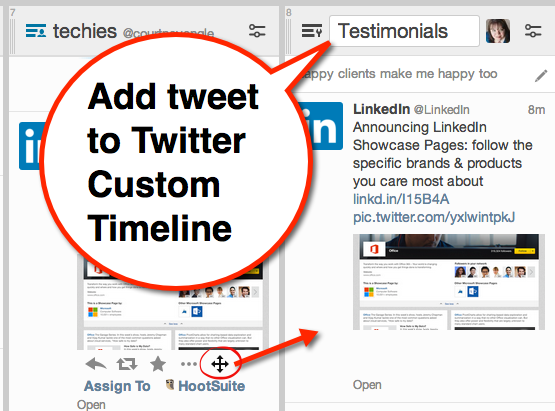The upper right corner of the image features a search bar containing the term "testimonials." Emerging from the search bar is a speech bubble outlined in red with the text "Add tweet to Twitter custom timeline." Adjacent to the search bar, a person's face is visible, characterized by dark hair and light skin.

Below this, there's content related to LinkedIn, which reads: "LinkedIn, @LinkedIn: Announcing LinkedIn showcase pages. Follow the specific brands and products you care most about," followed by a clickable link.

On the left side of the image, the word "Hootsuite" (spelled out as H-O-O-T-S-U-I-T-E) is prominent with arrows pointing in various directions around it, all circled in red. An additional arrow extends from this circle, guiding the viewer’s attention to the discussed LinkedIn link, which is displayed as "LinkedIn.in-15b4apick.twitter.com."